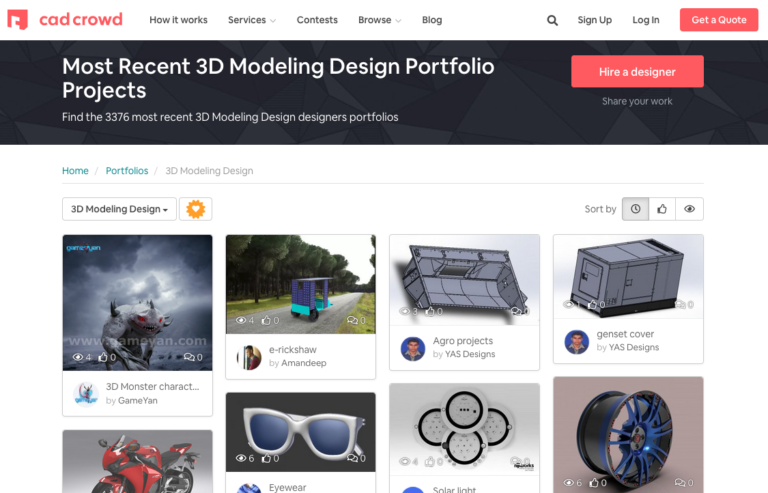In the upper left corner of the image, "CAD Crowd" is displayed in lowercase red text. Positioned to the right are navigation options: "How It Works," "Services," "Contests," "Browse," and "Blog." There is a magnifying glass icon next to these options, followed by "Sign Up" and "Log In." A prominent red rectangle features the text "Get a Quote" in white.

At the center of the image, the following white text is displayed: "Most Recent 3D Modeling Design Portfolio Projects" and "Find the 3,376 Most Recent 3D Modeling Design Designers Portfolios." Below, another red rectangle offers the option to "Hire a Designer," with the option to "Share Your Work" located beneath it.

The page is divided into sections labeled "Home," "Portfolios," and "3D Modeling Design." Underneath the "3D Modeling Design" section, two rows display various project thumbnails. The first row includes a gray monster titled "3D Monster Character," a large box titled "Gen Set Cover," and an image of a red motorcycle. The second row showcases a pair of silver sunglasses and a rim of a tire. Each thumbnail provides a glimpse into the diverse range of 3D modeling design projects available on the platform.